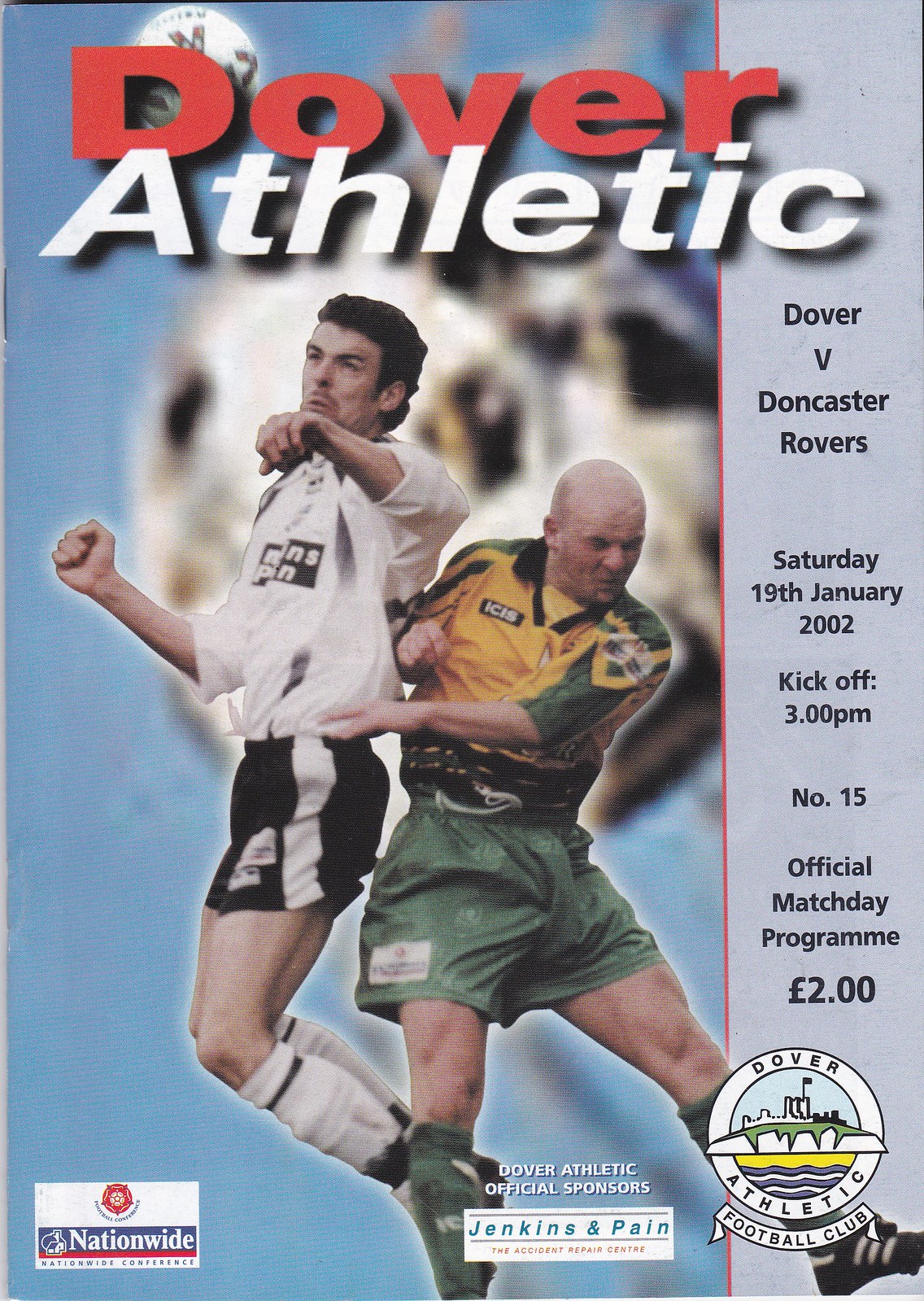This full-color cover of the official Dover Athletic match day program, priced at two pounds, features a dynamic image of two soccer players in action from an upcoming match against Doncaster Rovers. The game took place on Saturday, January 19, 2002, with kickoff at 3 p.m. prominently displayed. One player, with dark hair, leaps in the air wearing a white and black uniform, while the other player, who is balding, appears to be bracing for impact in his green and yellow jersey. The header reads "Dover Athletic," with a gray sidebar listing the match details: "Dover vs. Doncaster Rovers, Saturday, 19 January 2002, kickoff 3 p.m., number 15." On the lower part of the cover, logos for the Dover Athletic Football Club, Nationwide, and the club sponsors Jenkins and Payne are clearly visible, adding to the program's official and professional presentation.